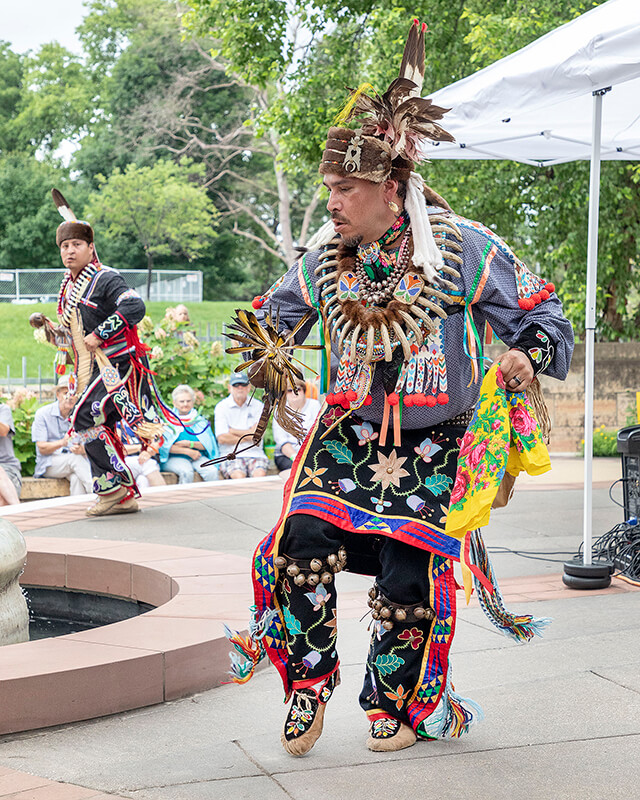The image depicts a ceremonial dance performed by two men in traditional Native American attire, with the focus on the central gentleman moving towards the left side of the frame. He is dressed in a strikingly colorful outfit, primarily featuring a blue shirt adorned with orange, green, and intricate multi-colored patterns. His headdress, made of white fabric and feathers, complements his pale skin, mustache, and partial beard, revealing an earring in his left ear. A prominent bone necklace adorns his chest, alongside a beaded necklace, with white fabric strips hanging below, each ending in a red ball.

His attire includes a skirt-like apron overlay with a central tan flower and green leaves, extending to floral and geometric patterns on his black pants. The pants are embellished with bells around the knees and terminate in traditional moccasins. In his right hand, he holds a noisemaker, while his left hand clutches a vibrant yellow handkerchief decorated with pink roses and various colors.

The background reveals the men dancing on a raised stone platform or patio, bordered by an audience suggesting an older community setting, possibly an old age home. Behind the seated audience are green lawns, flowering plants, and trees, with a patio umbrella visible on the man's right side. A minimal view of a circular inset or fountain can be seen, where the men perform their intricate, culturally rich dance.